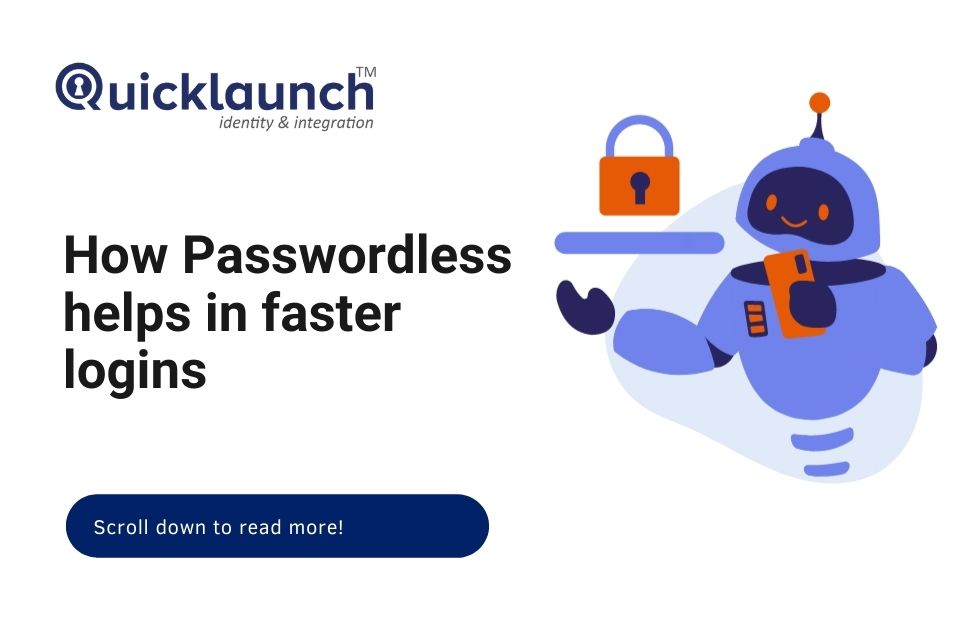The image designed for a website's quick launch page emphasizes themes of identity and integration. At the top, there is a black and white graphical symbol resembling a doorknob and keyhole, providing a visual reference to security and access. Above this symbol, the letters "TM" are displayed. Beneath the doorknob image, bold text reads "Quick Launch," followed by "Identity and Integration." Below this, larger black text states "How Passwordless Helps Faster Logins."

A blue column runs below the main text, featuring a call-to-action in white letters: "Scroll Down to Read More."

On the right side of the image, a robot is depicted holding a pink phone. The robot has a purple head and torso, although its lower body is represented by two simplistic lines. Extending from its hand, a gold lock with a purple top is prominently featured, alongside a horizontal purple line beneath it, symbolizing security and seamless access.